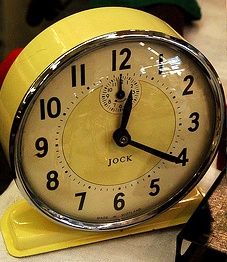The image displays a close-up of a retro-styled, antique-looking metal alarm clock sitting on a light-colored countertop, tilted at a slight diagonal angle with the lower left side closer to the viewer. The clock is predominantly bright yellow, featuring a chrome bezel around the front, which is covered by a reflective glass or plastic face. The main face of the clock is white, encircled by a yellow central ring, and it showcases bold, black Arabic numerals. An inset seconds dial with black numbers is situated just below the clock’s hands, which are both black and pointing to 12, indicating the time as approximately 12:20. The clock has a sturdy, flat metal stand at its base, designed to keep it upright. The brand name "Jock" is displayed prominently under the hands in the center of the clock face. The overall impression is one of a well-crafted, vintage yet modern table alarm clock, set in an indoor environment, with a hint of a brown table visible in the lower corner of the image.